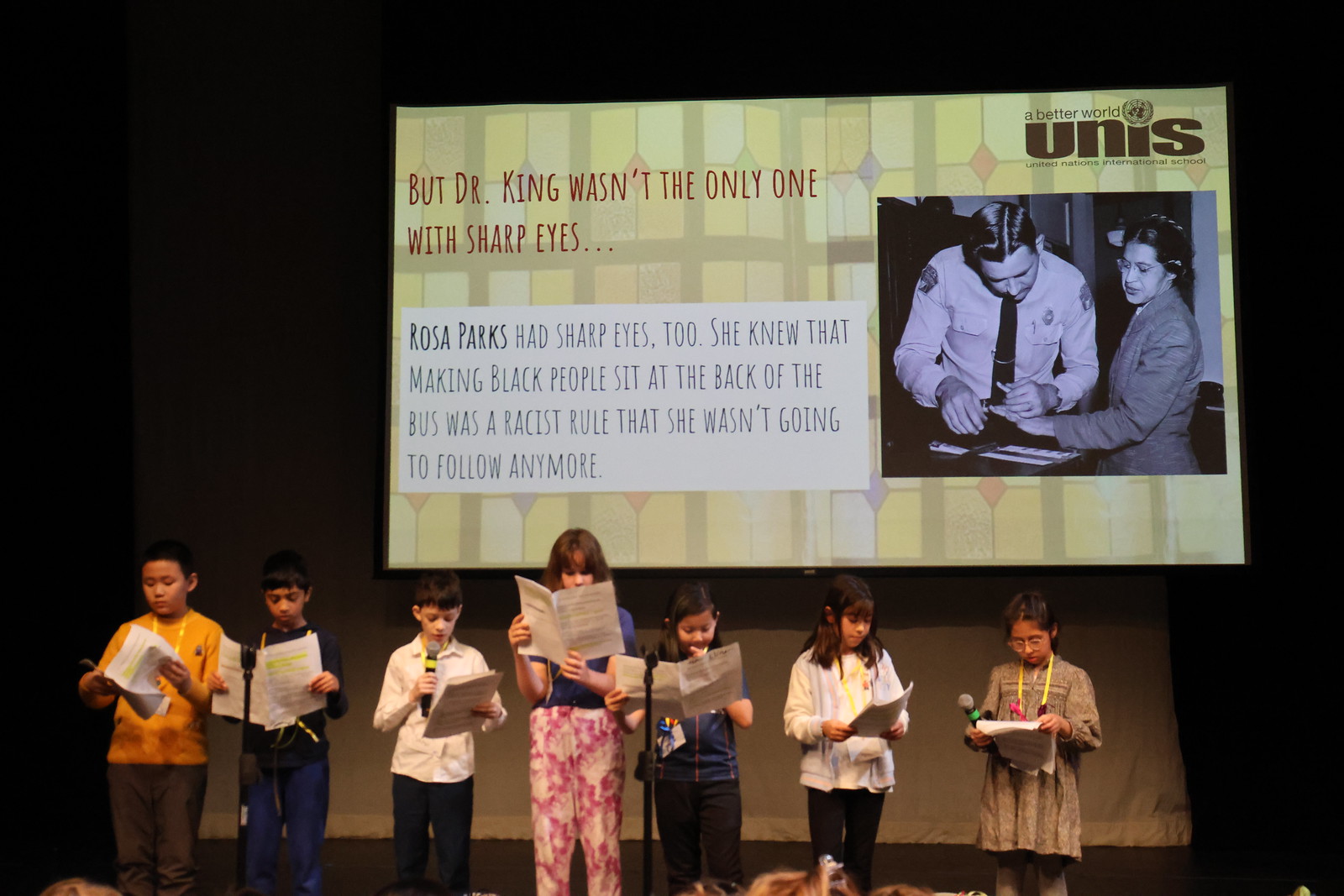This is a horizontally aligned rectangular picture of a school event at the United Nations International School featuring a group of seven children on a stage. There are three boys on the left and four girls on the right, each holding a piece of paper with yellow-highlighted sections. They are dressed nicely; one girl on the far right is wearing a brown dress, while the others are in various tops and pants. Some children are holding microphones or standing behind microphone stands—specifically, the second child from the left, the two girls in the middle, and the third boy from the left who is holding a microphone in his hand.

The background features a large rectangular screen with a projected image of Rosa Parks being fingerprinted by a police officer. The text in red reads, "Dr. King wasn't the only one with sharp eyes..." and in black text on a white background, it continues with, "Rosa Parks had sharp eyes too. She knew that making black people sit at the back of the bus was a racist rule that she wasn't going to follow anymore." The children appear to be reading or discussing their scripts, contributing to a presentation about Dr. King and Rosa Parks' roles in fighting racial injustice.